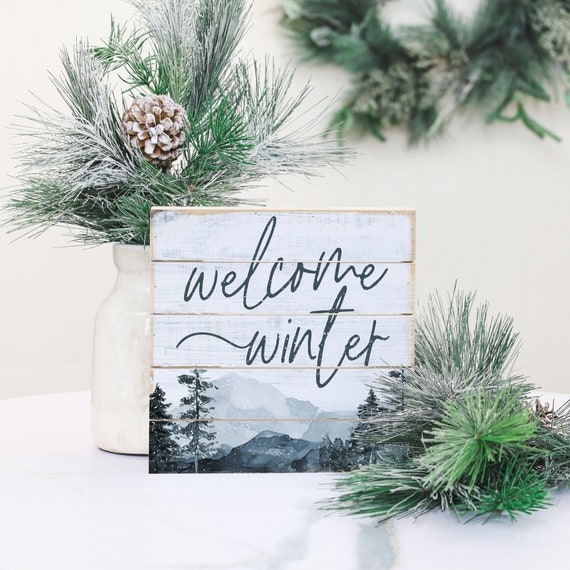This bright and inviting photograph captures a charming winter home decor scene. At the forefront is a square, slotted wooden sign painted white with rough edges that reveal its natural wood beneath. The sign features a whimsical "Welcome Winter" message in a swirly font, set against a mountain and tree winter motif. This piece rests on a white tabletop alongside what appears to be a farmhouse-style vase, reminiscent of an old milk jug, filled with pine needles and a pine cone. Additional pine needles are scattered around the base, enhancing the rustic feel. In the blurred background, a cream-colored wall hosts a green wreath, suggestive of evergreen or Christmas decor, bringing a festive touch to the composition. Every element, except for the wreath, is in sharp focus, contributing to the overall bright and cozy aesthetic of the scene.